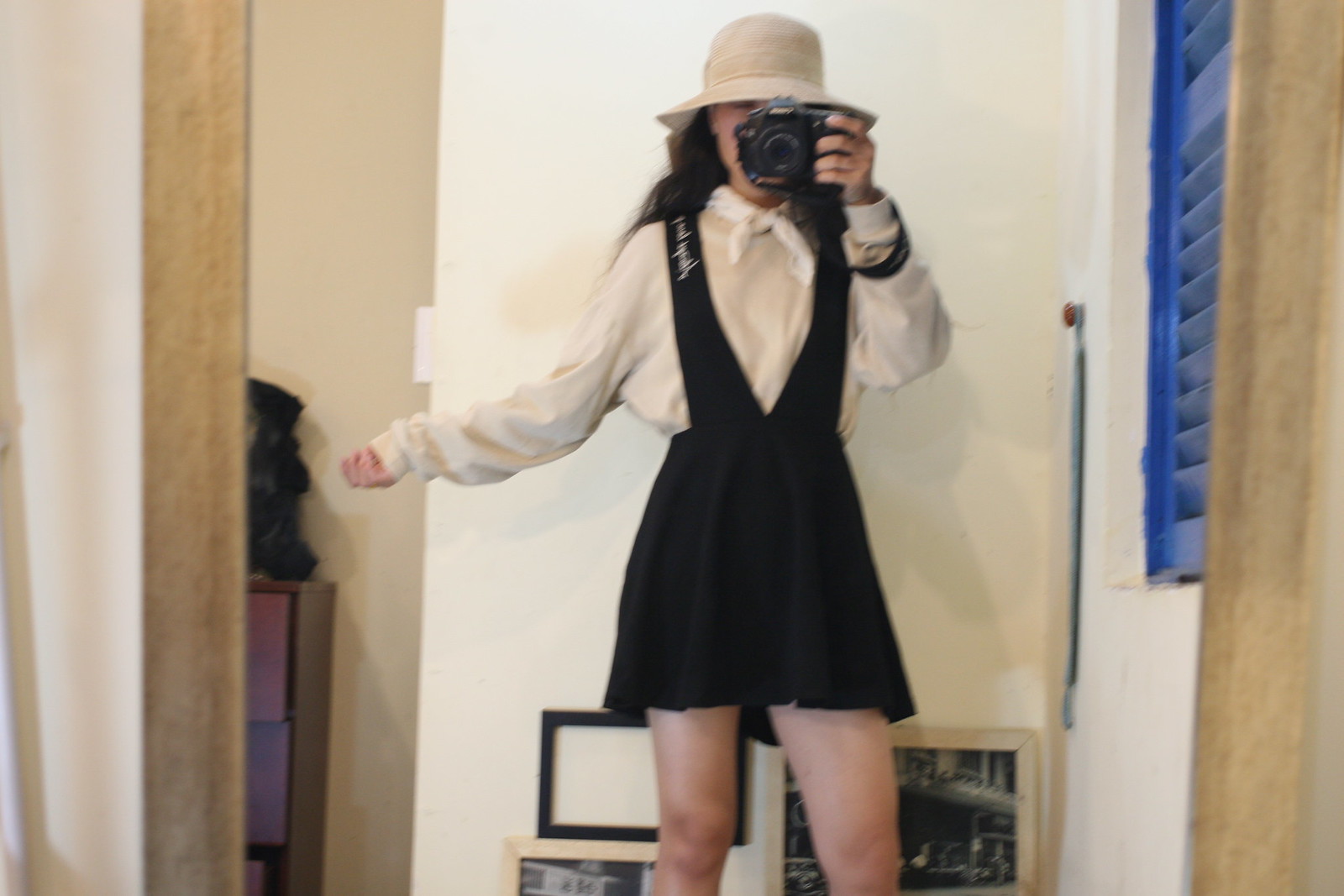In this detailed photo, a woman stands in front of an open door, visibly in a room that leads to another with beige walls. She is wearing a short black dress over a long-sleeved, fluffy white shirt, and accessorized with a big brown hat and a white scarf around her neck. Holding a black handheld camera up to her face with her right hand (appearing as her left hand due to the mirror's reflection), she takes a selfie, obscuring most of her face. Her left arm is outstretched to the side. The image, cut off at her knees, shows the mirror's light brown borders clearly, emphasizing the reflection. Surrounding her are blue window shutters and numerous picture frames scattered on the floor. A light switch is visible on the left side of the image, and part of a cabinet can be seen in the adjacent beige-walled room.